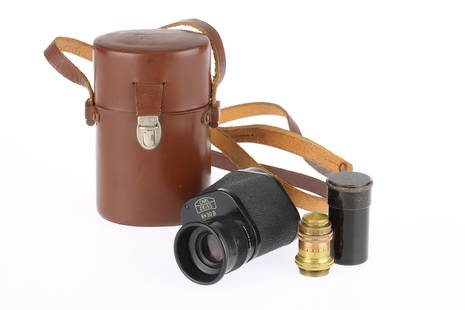The image displays a detailed arrangement of items centered around a single black binocular with a slightly reddish tinted lens and a textured, grippy housing. Accompanying the binocular are two additional small lenses, one black and one gold, designed to enhance the viewing capabilities. The setup includes a large brown leather carrying case with a silver clasp for secure closure, and a long strap for convenient neck wear. The case, which resembles a structured canister with a lid, provides storage for the binocular and its accessories, making it easy to carry and protect the equipment.